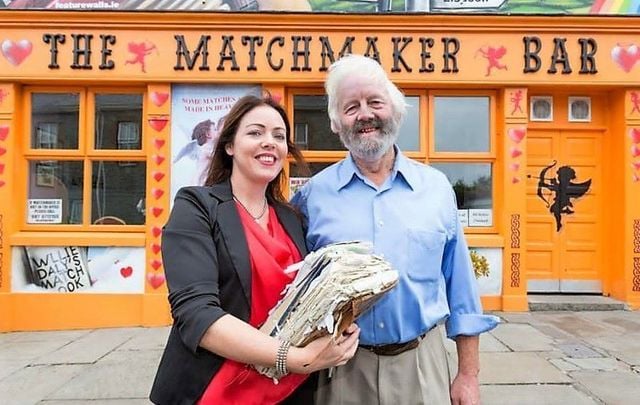In this vibrant photograph, an older man and a younger woman stand happily in front of the pumpkin-orange facade of the "Matchmaker Bar," a strip mall-style establishment. The bar's sign, adorned with a heart, the word "the," a reverse-faced cupid, and the word "matchmaker," catches the eye above the entrance. The charming front is decorated with playful red cupids and hearts, while a black cupid embellishes the double orange doors, which swing outward. The woman, possibly in her thirties or forties, with long black-brownish hair, dons a red shirt and a black blazer with rolled-up sleeves. She holds a large, tattered book filled with stuffed papers. Beside her is an older man with short white hair and a matching beard. He wears a light blue dress shirt with rolled-up sleeves, khaki pants, and a brown belt. The two smile warmly at the camera, possibly indicating their roles as proprietors of the bar. The bar's windows, set against the orange backdrop, carry additional text reading "Willie's Daily Matchbook," with further decorations including an illustration of a cupid kissing another cupid, accompanied by partially obscured red text. The scene is set on worn concrete tiles, suggesting a historical urban setting with cracks visible in the pavement.